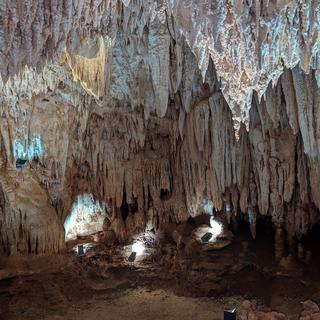This full-color photograph, slightly vertically rectangular, captures the interior of a cave characterized by numerous sharp, jagged stalactites hanging from its ceiling. These formations, mostly white with light gray and beige hues, sometimes have hollow centers and come to pointed ends. The cave’s ground is flat, compact, and covered with dark brown dirt and rock. Five man-made spotlights are strategically placed: three towards the bottom center, one in the left middle, and one at the bottom right corner. These bright white spotlights, drilled and inserted into the cave walls, illuminate the striking stalactites above and create dramatic contrasts between the well-lit upper area and the darker lower ground. The photograph highlights the cave's rugged beauty and utilizes artificial lighting to enhance the visual impact, depicting an eerily serene subterranean scene devoid of any human presence.